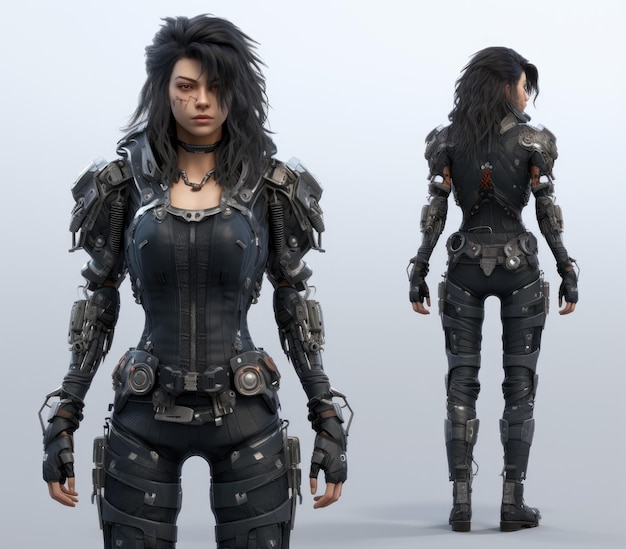The image portrays a digitally created or AI-generated character design, featuring a young female character with two perspectives: a close-up front view on the left and a smaller back view on the right. Both views emphasize a consistent and detailed military-style black outfit equipped with various metallic elements. Her black hair extends shoulder-length, appearing disheveled and spiky, enhancing her intense and serious demeanor. The character's face is pale with noticeable facial scars, adorned with a black band and necklace. 

Her attire includes armored shoulder guards, a tight bodice with metallic buckles, and leg holsters, contributing to the overall combat-ready appearance. Her arms are distinctly robotic, showcasing wires, hinges, and metal components that blend seamlessly into her outfit. This robotic aspect extends to her legs and shoes, all exhibiting a metallic, mechanical design. The background is a neutral grey, highlighting the intricacies of her elaborate ensemble, which is consistently depicted across both the front and back profiles.